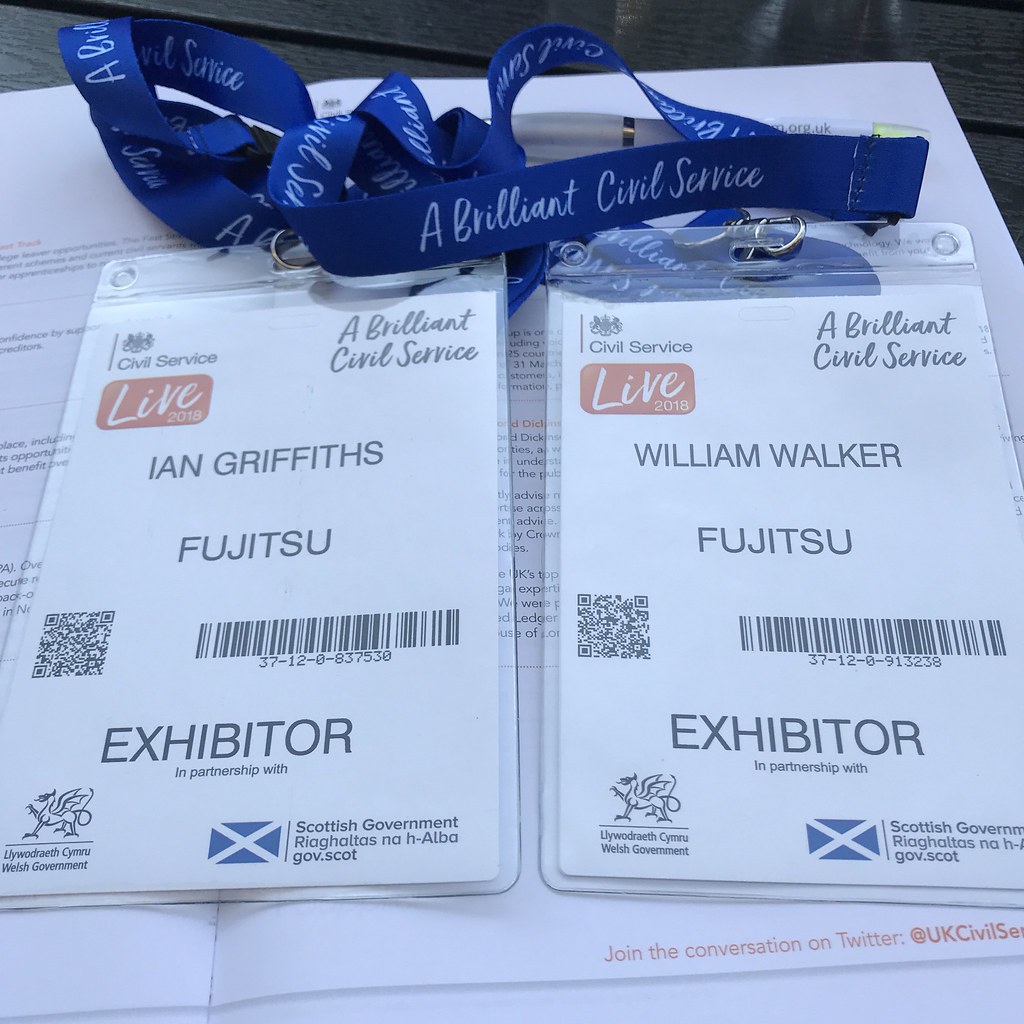The image depicts two identical ID name tags placed side by side on an open booklet, which is resting on a black surface. Each name tag is encased in a clear plastic holder and attached to a blue lanyard bearing the words "A Brilliant Civil Service" in white. The lanyards have gold-colored rings connecting them to the plastic holders.

The left ID tag displays "Ian Griffiths," while the right ID tag reads "William Walker." Both tags feature the same layout and design elements. At the top left corner, there's a logo followed by the words "Civil Service Live 2018" in white font on a red rectangular background, and the phrase "A Brilliant Civil Service" at the top right corner in grey font. Below the names, "Fujitsu" is mentioned. Both tags include a QR code on the left and a barcode on the right, with unique numbers beneath each barcode.

At the bottom center of each tag, the word "Exhibitor" is prominently displayed in large uppercase letters, followed by "in partnership with." The left bottom corner features the logo and words "Llywodraeth Cymru Welsh Government" with an icon of a mythical dragon, while the right bottom corner has a blue-and-white flag icon and the text "Scottish Government," along with “gov.scot.”

Beneath the ID tags, on the bottom right corner of the booklet, there’s a footnote in orange text prompting viewers to "Join the conversation on Twitter @UKCivilService."